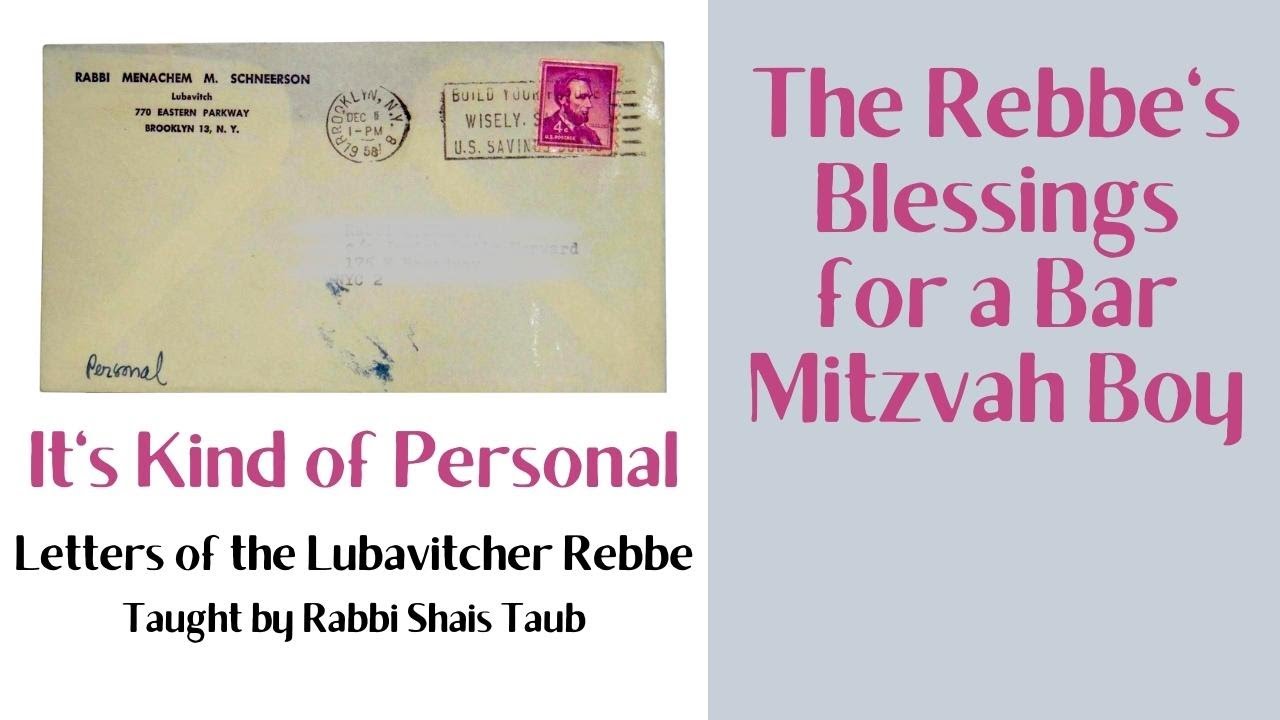The image collage features a white background and is divided into sections. In the top left corner, there is an image of a mailed envelope addressed to Rabbi Menachem M. Schneerson, also known as the Lubavitcher Rebbe. The return address is listed as 770 Eastern Parkway, Brooklyn, New York, and the envelope bears a postal stamp indicating it has been processed by the post office. Directly below the image of this envelope, there is a text that reads: "The kind of personal letters of the Lubavitcher Rebbe, taught by Rabbi Shais Taub." This likely indicates that the image is part of an advertisement for a series or lecture about the personal correspondence of the Rebbe. On the right, occupying the right half of the collage, there is a gray text box with pink font stating: "The Rebbe's blessing for a Bar Mitzvah boy," suggesting that the personal letter in the envelope is a blessing from the Rebbe intended for a Bar Mitzvah boy.